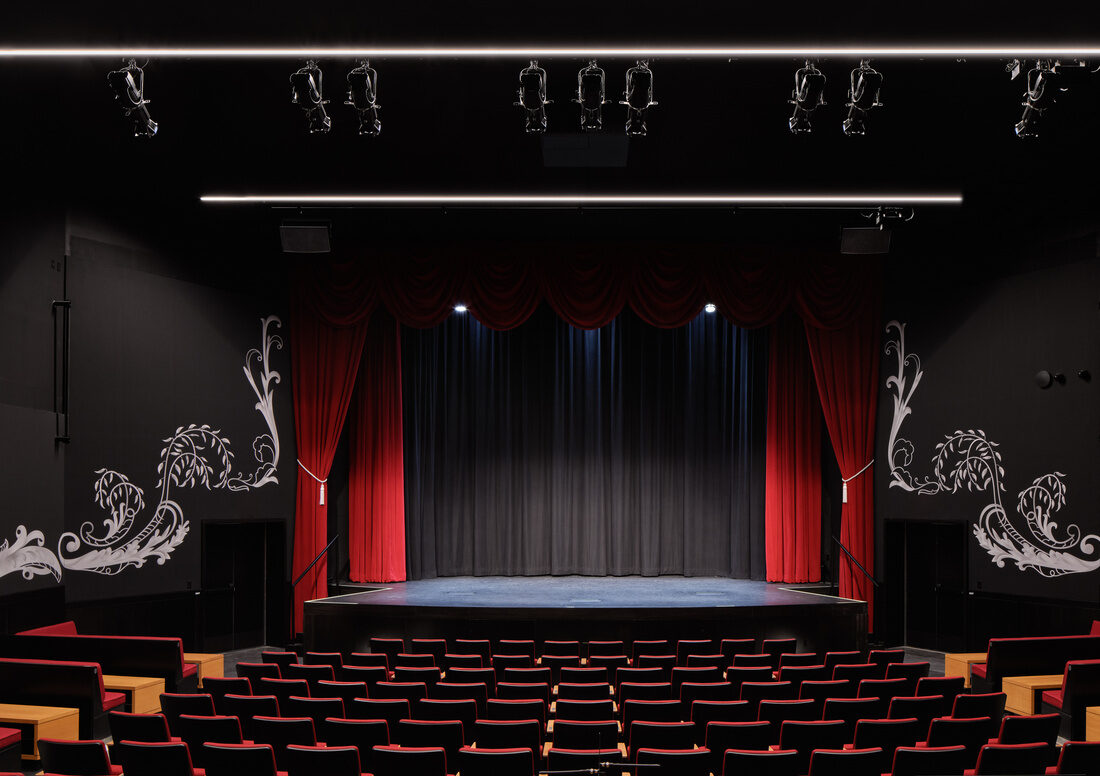The image depicts a theater set up for live performances, featuring predominantly black walls adorned with a white floral pattern. A black curtain forms the backdrop of the stage, which is flanked by red curtains draped from both sides, held back by white tassel ropes. In the center stage, two lights shine down from above. The seating consists of numerous rows of red theater chairs, with a couple of chairs positioned in the middle of the stage and longer formations of chairs arranged on either side for the audience. At the top of the stage, around nine lights are visible, casting a glow downwards, and below them, speakers are aimed toward the audience. Access stairs are present on either side of the stage, enhancing its accessibility. The overall ambiance suggests a venue well-prepared for live theatrical performances, emphasizing the intricate balance between elegance and functionality.